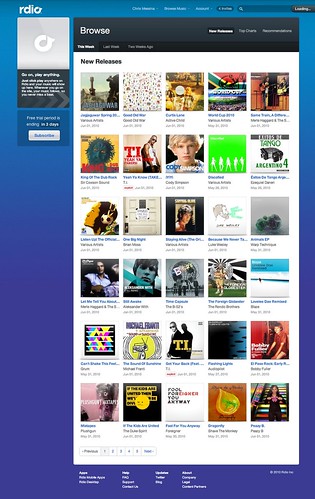The image is a screenshot taken from a website that resembles Spotify or a similar music streaming service. The background is a gradient of purplish-blue, predominantly towards the upper left corner. In this area, the word "RDIO" is prominently displayed in white text, presumably an abbreviation for "radio."

Towards the center-right, there is a series of white buttons intended for dropdown menus, though the text is too fine and blurry to read clearly. Adjacent to this is a search bar.

On the far right, there is a black section featuring the word "LOADING" in white text. Beneath this, within an area designated for album artwork, there is only a gray square present. Moreover, there are two additional squares: one black with unreadable white text and another in darker purple also with indistinguishable white text.

To the right of the supposed album artwork, a significant black navigation panel is visible. This panel clearly displays the options "BROWSE," "New Releases," "Top Charts," and "Recommended" in white text.

Below this, a large white section showcases an extensive collection of album covers, arranged in six rows of five. Each album is accompanied by text in white or blue, but the specific details are not discernible.

At the very bottom of the screenshot, there is more white text likely containing links for contact information, home navigation, and other standard footer content, although this text is also too blurry to read.